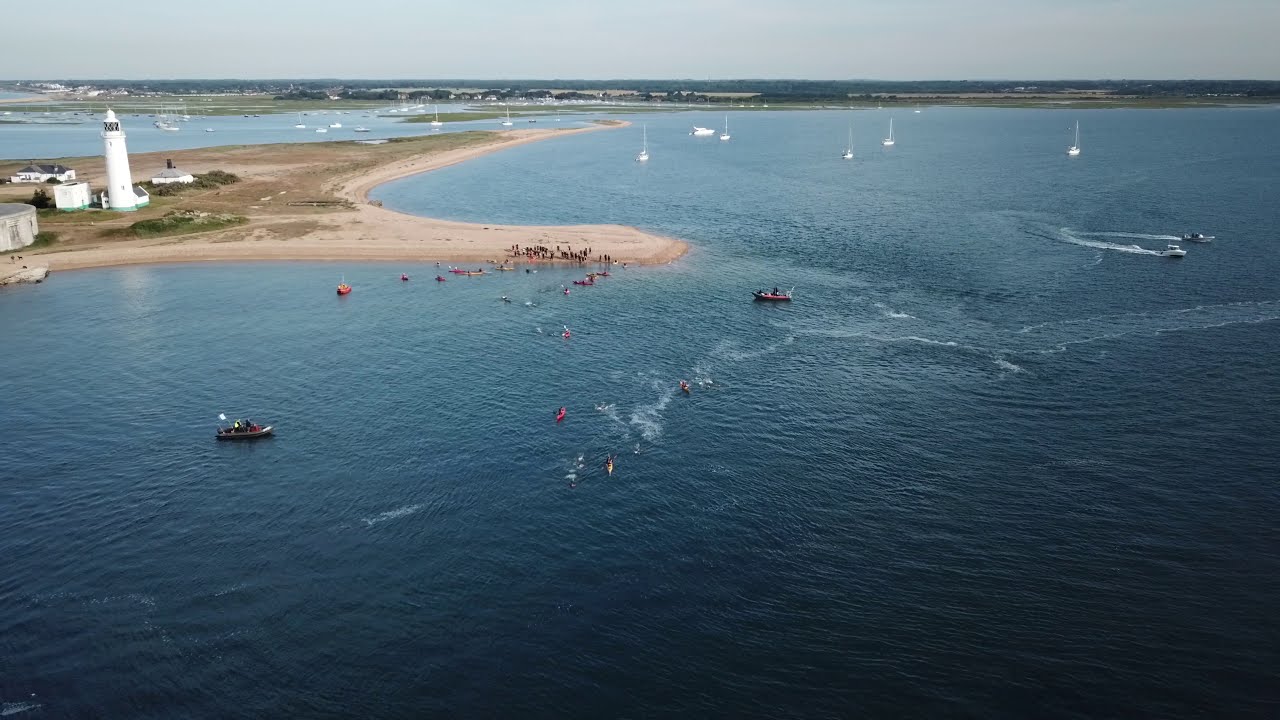This overhead image, likely taken from a drone or plane, captures a wide expanse of coastal water with a distinctive sandy peninsula in the upper left corner. The peninsula, possibly part of a larger landmass, features a prominent white lighthouse surrounded by a few small buildings, and it houses a group of people standing near the coast. The horizon, positioned near the top eighth of the image, is dotted with sailboat masts. In the upper right, two boats or jet skis create visible wakes on the water's surface. Scattered throughout the mid and lower thirds of the image are additional boats, including sailboats and motorboats, alongside more groups of people both on the beach and in the water. The scene is framed by a partially cloudy sky and a backdrop of trees, further enhancing the natural beauty of this coastal area.